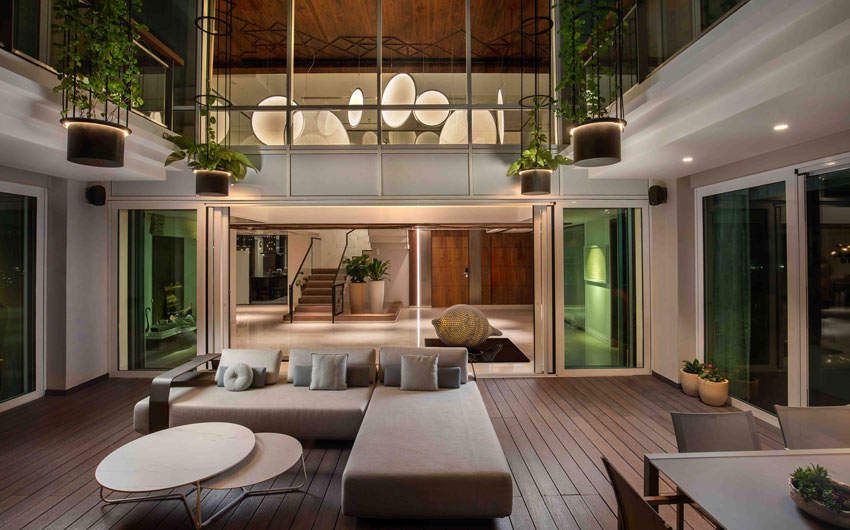The image depicts a spacious and ultra-modern living and dining area spanning two levels. The lower level features an L-shaped sectional sofa with three sets of pillows and an armrest on its right side, all situated on a floor with grey wooden planks. In front of the sofa, there is a stylish round coffee table with a smaller round table partially tucked underneath. The living room flows seamlessly into the dining area, which is situated in the lower right-hand corner and features a modern table paired with grey chairs.

Flanking the room are glass doors on both sides, creating a bright and airy atmosphere, although the outside appears to be dark. In front of the right sliding glass door, several planter pots can be seen. The walls of the room extend up to the ceiling, which is made of wood and adorned with various sized hanging circular lights. Additionally, plants cascade from the second floor, with one large planter and other pots hanging down with integrated lighting.

A staircase with two large planters leads to the second floor, which is visible through the expansive glass wall. The upper level continues the modern aesthetic with its hanging lights and additional greenery. Overall, the space cohesively blends sleek, modern furnishings with a bright, open architectural design.